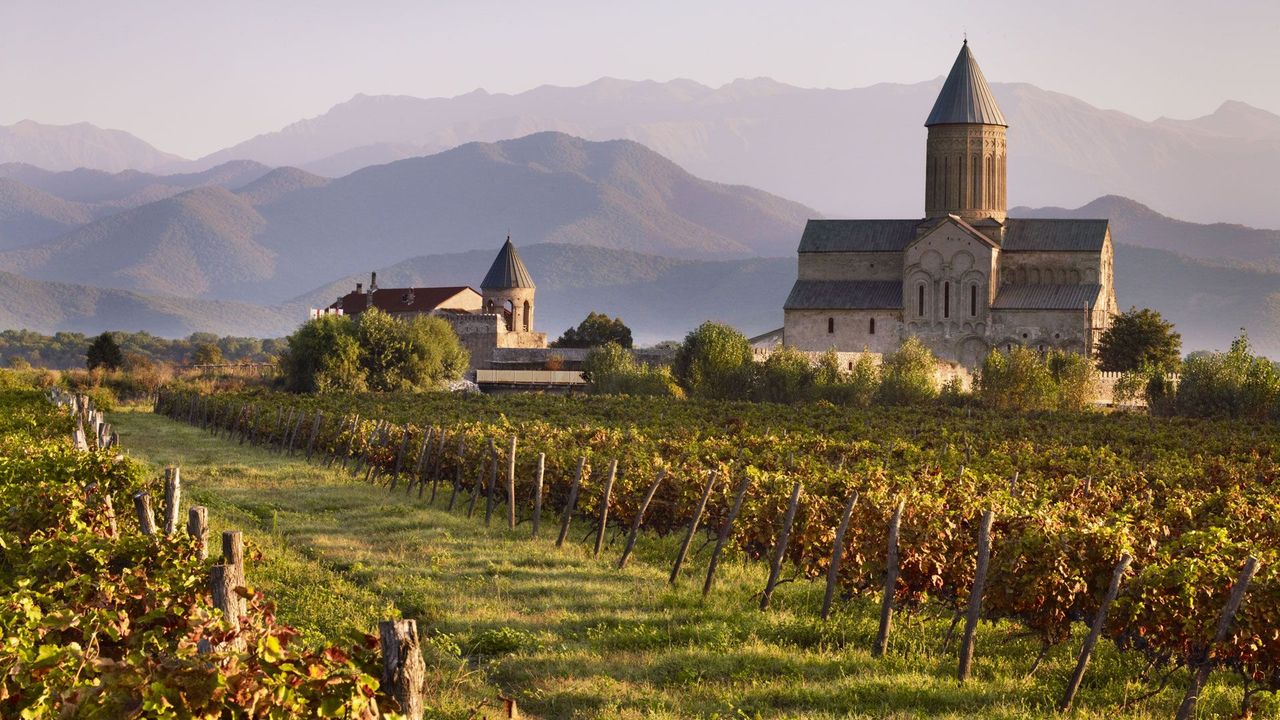The photograph captures a picturesque European countryside at dusk, characterized by an ethereal sky and a verdant mountain range in the background, cloaked in a misty, smoky silhouette. Prominently, two stone buildings dominate the scene: a substantial church or castle-like structure with a multi-layered roof and a smaller steepled building, both exhibiting classic architectural elegance. The foreground is marked by a vibrant, meticulously planted row of flowers or possibly grapevines suggesting a vineyard, with a well-trodden, green grassy path weaving through. The entire landscape conveys a serene, timeless beauty, blending historical charm with pastoral serenity.